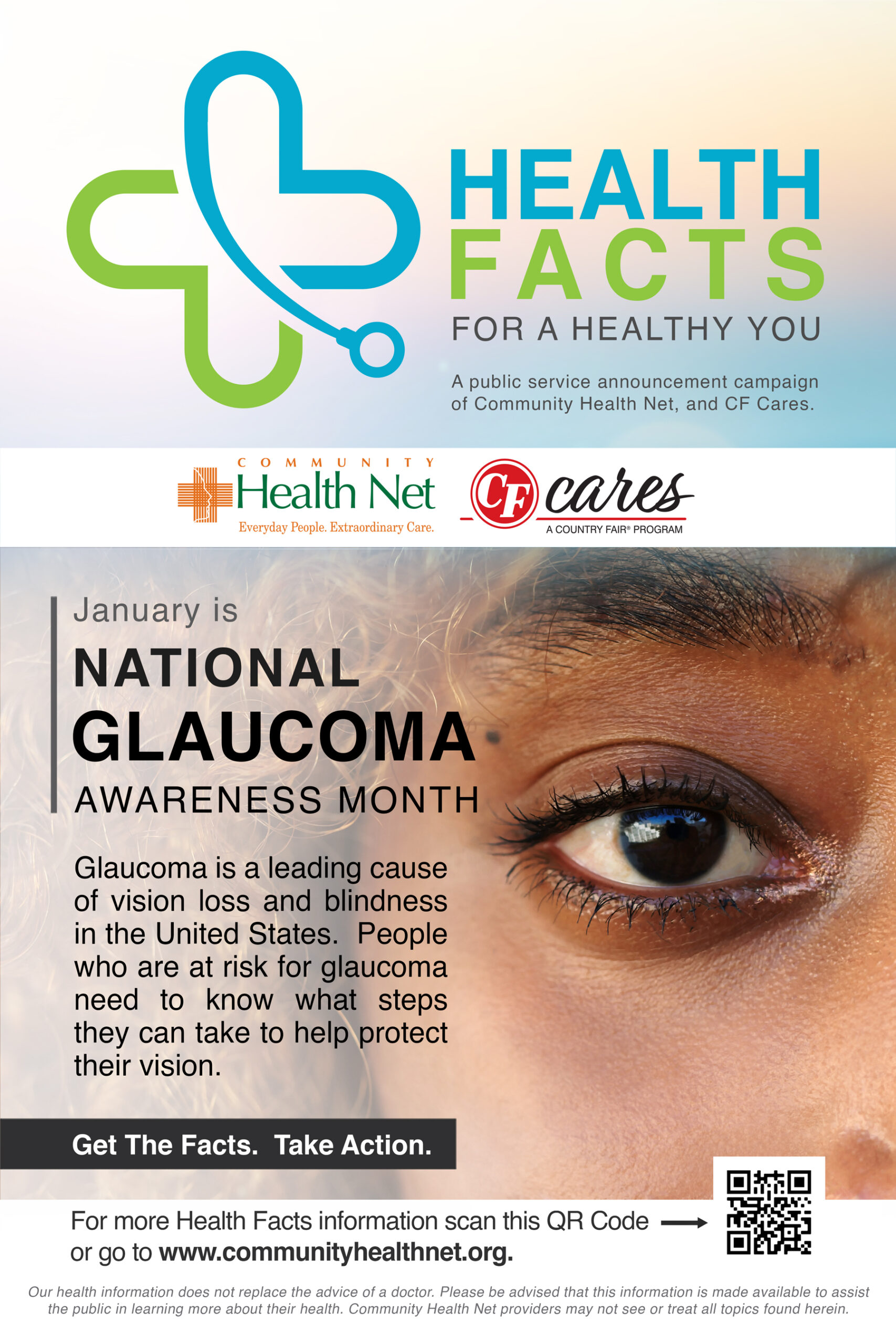This is a detailed public service announcement poster for "Health Facts for a Healthy You," a campaign by Community Health Net and CF Cares. The vertical, portrait-oriented poster is split into two halves. The top half features a blue and green cross logo, with "Health" in blue and "Facts" in green. Below the logo, the text reads: "For a Healthy You, a public service announcement campaign of Community Health Net and CF Cares,” accompanied by their respective logos.

The lower half of the poster focuses on raising awareness for National Glaucoma Awareness Month. It includes a close-up image of a woman's eye—the upper left portion of her face is visible, including her dark eye, dark eyelashes, and a blonde streak in her hair. She has darker skin and is staring directly into the camera, with a reflection visible in her eye. To the left of her image, black text reads: "January is National Glaucoma Awareness Month," followed by a descriptive paragraph about glaucoma, its risk factors, and the importance of taking steps to protect vision. At the bottom, there is a URL and a QR code for more information.